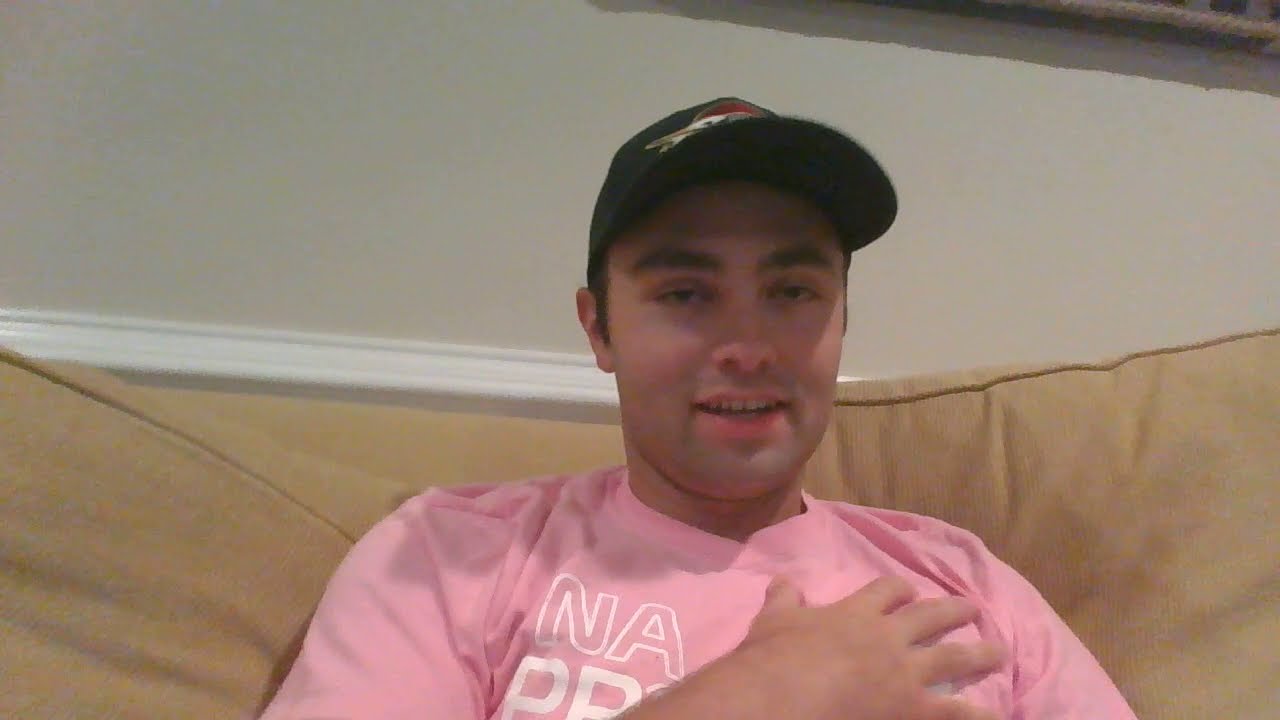The photograph features a young man, likely in his early 20s, sitting on a light brown couch against a grayish-brown wall with white wainscoting. He has a fair complexion, dark hair, bushy eyebrows, and dark eyes, possibly brown. He is clean-shaven and wears a black baseball cap with an indiscernible image on the top. The young man is dressed in a pink t-shirt with white-outlined letters, partially reading "N A," followed by a possibly obscured "P," "B," or "R." His right hand is placed over his heart. He sits centered in the image, looking directly at the camera with a subtle smile. In the top right corner of the photo, an object casts a shadow that extends from two-thirds of the way across to the edge of the frame, adding a touch of intrigue to the otherwise straightforward setting.